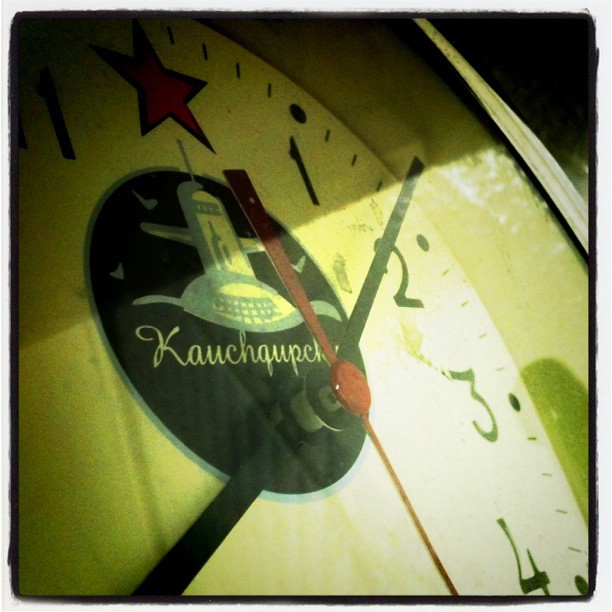This photograph is a close-up of a vintage wall clock taken at an artistic angle. The clock's face is visible only from the lower left to the upper right section, prominently showcasing the bold black numbers 1, 2, 3, and 4 against a yellowish-tan background. A striking red star replaces the number 12 at the top center of the clock. Beneath the star, a black circular disc features white cursive text, partially obscured by one of the black hour/minute hands, with distinct lettering like "K-A-U-C-H-Q-U-P-C-H." Above this text, there is a blue and white design resembling a spaceship or rocket. The clock hands are black, with the hour hand pointing towards the 2 and another hand extending towards the lower left corner, while a red second hand moves from the star towards the lower right. The overall image is reminiscent of 1950s diner art or a cowboy-themed decor, and includes a bright spot indicating a light source in the bottom right corner. A thin black line borders the clock, which itself is framed by a white border, enhancing its artistic presentation. The background and framing suggest the clock has depth, and the highlighted details further evoke a sense of nostalgia.